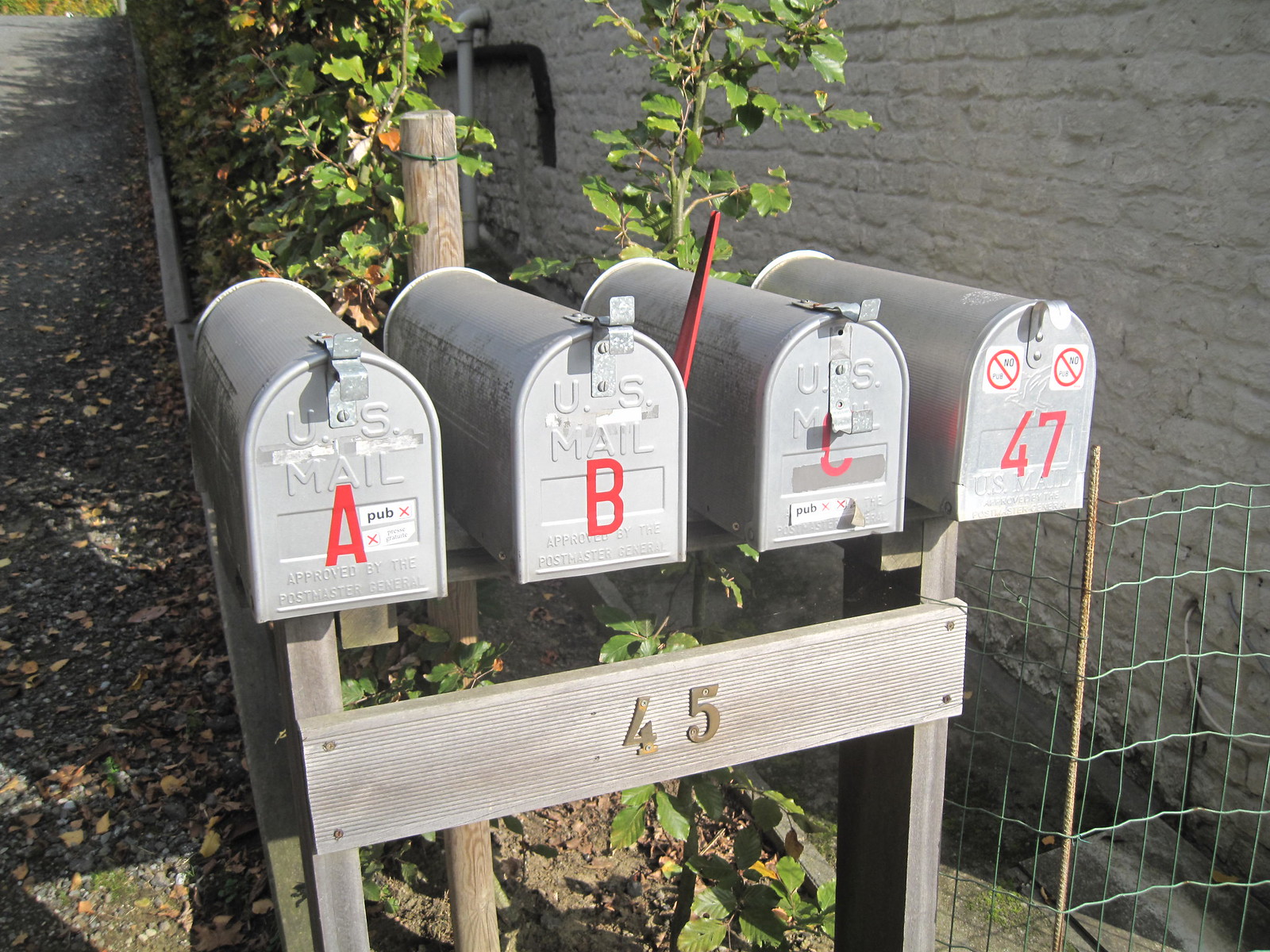This outdoor color photograph captures a set of four silver mailboxes mounted on a single wooden stand, positioned in what appears to be an apartment complex. Each mailbox prominently features "U.S. MAIL" and "Approved by the Postmaster General" embossed on the front. They are labeled with red letters and numbers: the first is marked A, the second B (with its red flag upright indicating mail to be picked up), the third C, and the fourth 47, which additionally bears two round labels with diagonal lines through them. The wooden stand that supports these mailboxes displays the number 45 in gold. Behind the mailboxes, there is a black, possibly asphalt area with scattered dry leaves, resembling a driveway. A holly bush and a white cable line against the backdrop of a white brick wall are also visible. Nearby, a section of metal wire fencing suggests restricted access.